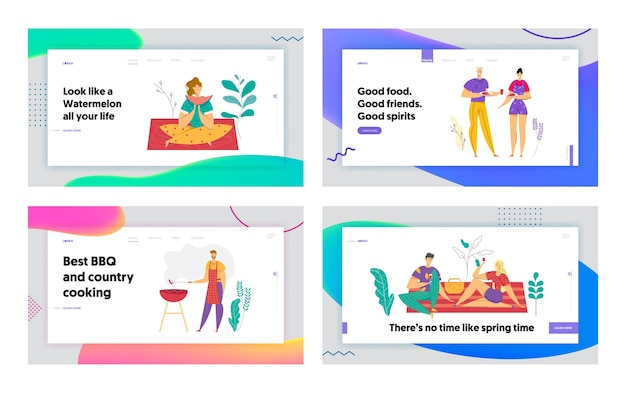The image is divided into four rectangular sections arranged in a 2x2 grid. Each section has an outline primarily in gray, with distinct colors and patterns embellishing the interiors.

In the upper left-hand quadrant, green dominates the scene with blotches, zigzag lines, and circles. It features a caption that reads, "Look like a woodman all your life," illustrating a person with a red apron, grilling on a red barbecue set amidst green foliage. Below the man, another caption states, "Best BBQ and country cooking."

The upper right-hand quadrant showcases hues of purple with similar zigzag lines and blotches. This section bears the phrase, "Good food, good friends, good spirits," depicting a man holding a plate of food and a drink, conversing with a woman who also holds a plate of food.

In the lower left-hand corner, pink is the primary color, accompanied by yellow blotches, dots, and swirls. This scene focuses on two people enjoying a picnic, seated on a red and orange striped blanket with a yellow picnic basket, surrounded by leaves. It carries the sentiment, "There's no time like springtime."

The lower right-hand quadrant is predominantly blue, highlighted with green blotches and zigzag lines. This part does not have additional descriptive content but maintains the thematic consistency of nature and outdoor activities. 

Overall, the image captures a vibrant collage of seasonal, outdoor activities focused on food, companionship, and the beauty of spring.